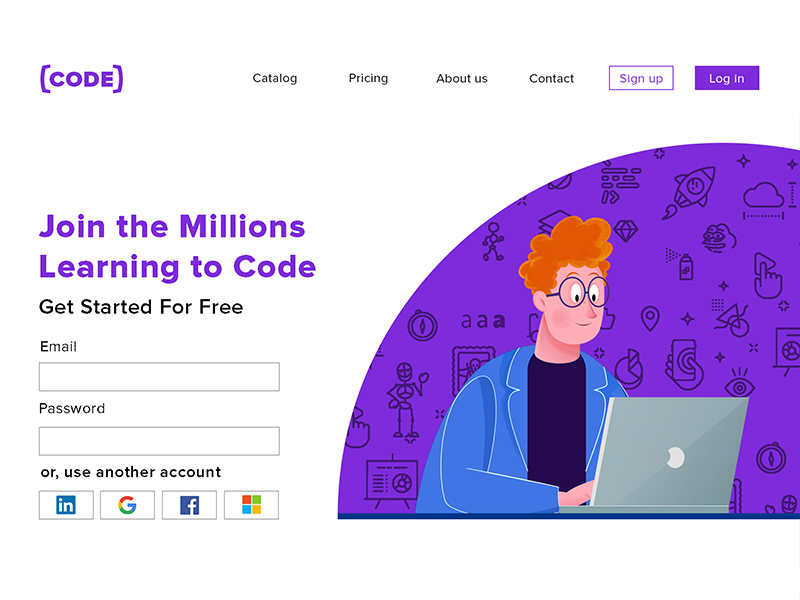The landing page for the coding website features a prominent logo at the top displaying the word "CODE" in all caps, framed within brackets and rendered in bold purple letters. Directly above, a navigation menu is aligned to the right, offering links to "Catalog," "Pricing," "About Us," and "Contact." Accompanying the menu are sign-up and login buttons, with the "Sign Up" button outlined in purple and featuring purple text, and the "Login" button solid purple with white text.

Beneath this, a large, left-aligned headline in striking purple font invites users to "Join the Millions Learning to Code." Following this, a subheading encourages them to "Get Started for Free," accompanied by fields for email and password entry, or alternative login options through LinkedIn, Google, Facebook, or Microsoft.

To the right side of the page, a whimsical graphic depicts a cartoonish male figure characterized by reading glasses, an open laptop, a purple shirt, a blue blazer, and orange hair. A partial circular graphic, resembling a pie chart, surrounds him from behind and extends off the edge of the image.

At the bottom of the page, a blue horizontal line runs across, below which several darker purple icons are displayed, including a rocket ship, spray can, map, mobile phone user, eyeball, wall clock, robot, skeleton, pie chart on an easel, and clouds with measurement tools. These icons symbolize the diverse problems that coding aims to solve.